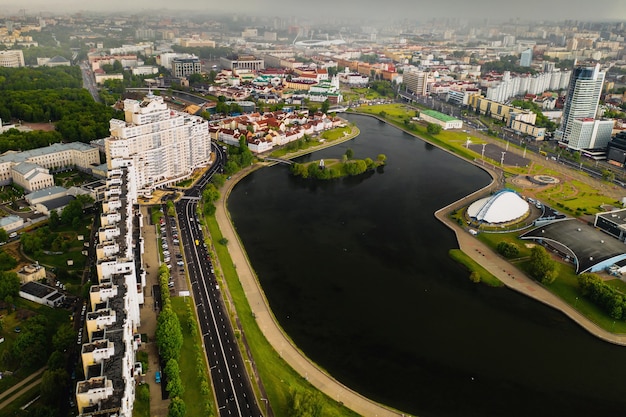This aerial color photograph captures a sprawling cityscape along a curving, dark river, likely taken from a drone or traffic helicopter. The waterfront boasts wide, concrete walkways bordered by a green strip, offering scenic vistas along the water’s edge. Several small islands dot the river, adding a picturesque element. Dominating the riverbanks are diverse structures: to the left, a four-lane divided boulevard runs parallel to a massive white facaded building, possibly a hotel, towering up to 20 stories high. Adjoining it are rows of smaller white buildings that extend towards the horizon. On the right, a notable white-domed building stands out amid a mix of skyscrapers and lower structures, capturing the city’s architectural diversity. Further right, a stadium or power plant sits prominently by the river, contributing to the urban hustle. The scene stretches endlessly with a hazy, somewhat polluted sky draping the horizon, emphasizing the city's vastness. Sparse traffic is visible on the boulevard, and the river's black water contrasts sharply with the greenery of trees and grass scattered throughout the urban expanse.